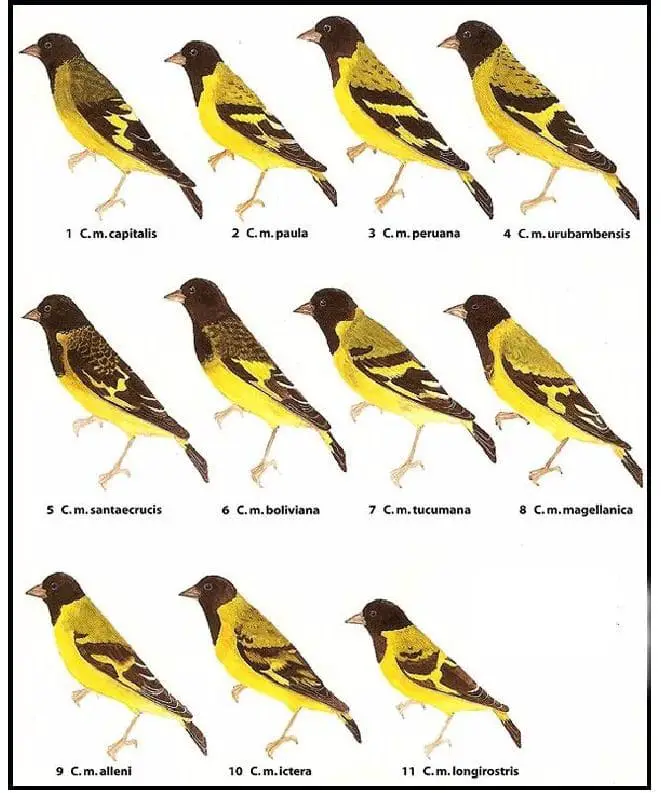This detailed illustration showcases eleven distinct subspecies of goldfinches, each meticulously labeled and numbered from one to eleven. The artwork, set against a white background and framed with a black outline, highlights each bird perched with one leg raised. These finches, primarily characterized by their black heads and vivid yellow bodies, exhibit subtle variations in their black and yellow feather patterns, particularly noticeable at the top of their wings and tails. Each bird is identified with a scientific name starting with "C.M." followed by a unique suffix, such as Capitalis, Perunua, and Paula. Despite their slightly varied sizes and designs, all finches share common features like tan-colored feet, yellow beaks, and a harmonious blend of black and yellow plumage, illustrating the diversity within this species.